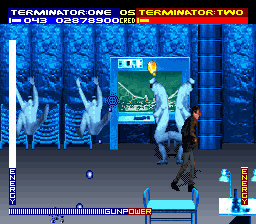Screenshot captured from a video game depicting a tense conflict unfolding in a bio lab. At the center of the scene, a bio lab cabinet is the focus of a skirmish; two characters donned in white protective suits and masks appear to be breaking into the cabinet, with visible signs of shattered glass suggesting forceful entry. Nearby, two workers are seen collapsing, possibly as a result of the attack. The backdrop features a blue glass chamber, adding to the futuristic and sterile environment.

In the foreground, a character dressed in street clothes—a Caucasian man wearing a brown coat, gray pants, and black shoes—is captured from the side as he walks away from the chaotic scene, hinting at his possible involvement or escape. The lab's floor is light gray, scattered with additional equipment including a lab cart, a table with several lamps, and a microscope, all of which emphasize the setting's scientific nature.

Overlaying the scene, there is text at the top of the screen in white letters divided by a horizontal blue and red bar, displaying "Terminator 1-0-5 Terminator 2" along with a series of numbers and letters: "I-0-4-3-0-2-8-7-8-9-0-0 C-R-E-D." A vertical bar on the left-hand side shows a measurement labeled "Energy," currently about a fifth full. At the bottom, another monitor indicates "Gunpower," nearly full. Lastly, a vertical guide with a red background and yellow letters on the right-hand side also displays the word "Energy," contributing to the game's interface.